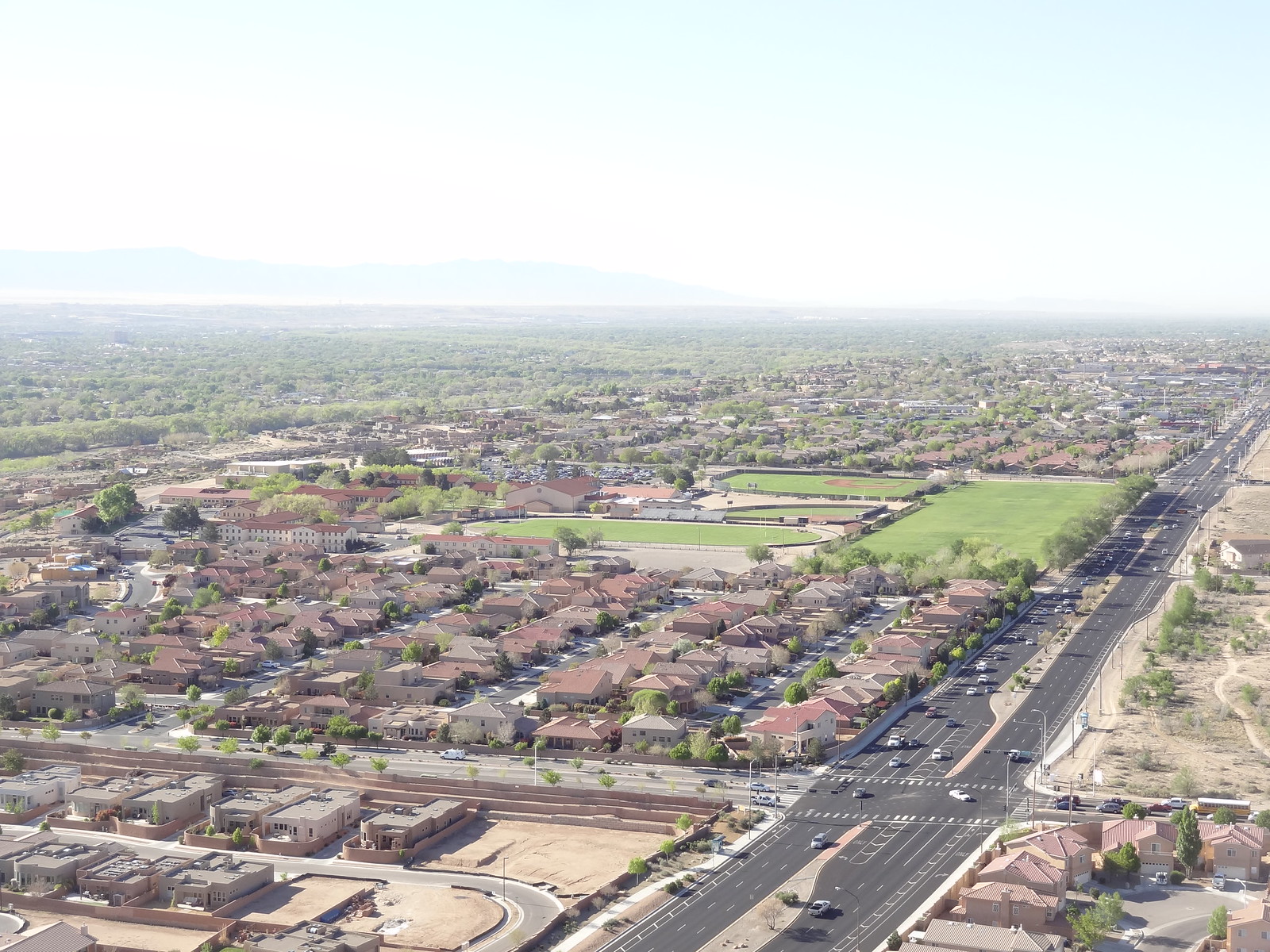The aerial photograph captures a sprawling suburban neighborhood, likely taken by a drone from a significant height. The landscape is predominantly flat and exhibits a dry, arid environment. In the center of the image, there is a grid-like arrangement of houses, meticulously aligned within what appears to be a square-shaped area. Interspersed among the residential zones are patches of lush greenery, which could be parks or undeveloped plots of land. To the right side of the image, a highway cuts through the scene, providing a stark contrast to the orderly residential expanse. The thorough detailing of urban planning and natural spaces offers a dynamic view of suburban living from a bird's-eye perspective.